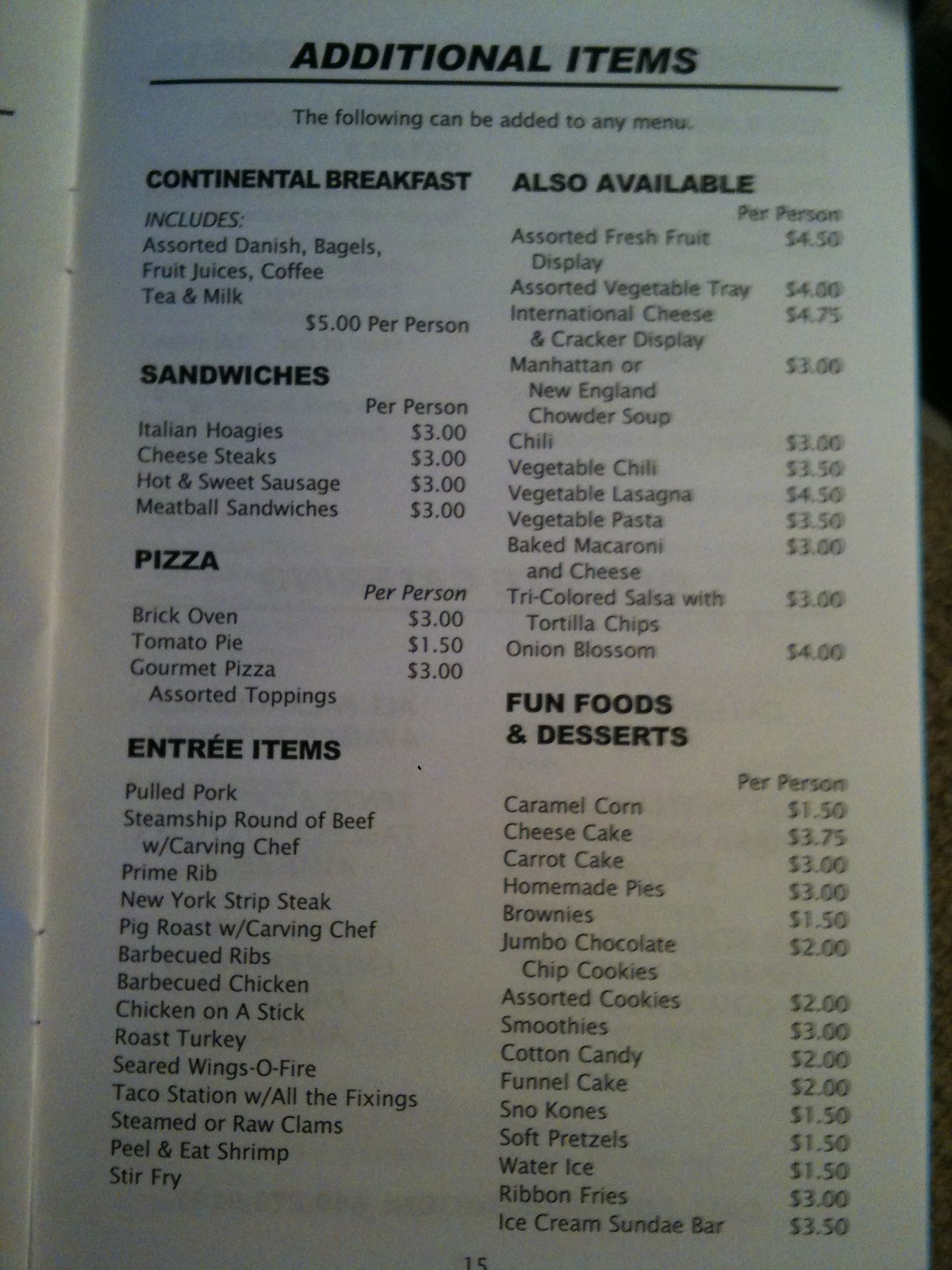This is an image of a detailed restaurant menu, potentially from a catering service, presented on slightly discolored whitish paper with black text. The menu is bound on the left, suggesting it could be part of a booklet, magazine, or book. 

At the very top, the menu features the heading "ADDITIONAL ITEMS" in all caps, underlined with a thick line. Below, it states: "The following can be added to any menu." 

The food items are organized into several sections, each with bolded, all-caps headings:

1. **CONTINENTAL BREAKFAST:**
   - Includes Danish, bagels, fruit juices, coffee, tea, and milk for $5 per person.

2. **SANDWICHES:**
   - Italian Hoagies: $3 per person
   - Cheese Steaks: $3 per person
   - Hot and Sweet Sausage: $3 per person
   - Meatball Sandwiches: $3 per person

3. **PIZZA:**
   - Brick Oven: $3 per person
   - Tomato Pie: $1.50 per person
   - Gourmet Pizza: $3 per person
   - Assorted Toppings

4. **ENTRÉE ITEMS (Also Available):**
   - Pulled Pork
   - Steamed Ship Round of Beef with Carving Chef
   - Prime Rib
   - New York Strip Steak
   - Pig Roast with Carving Chef
   - Barbecued Ribs
   - Barbecued Chicken
   - Chicken on a Stick
   - Roast Turkey
   - Seared Wings of O'Fire
   - Taco Station with All the Fixings
   - SLW (Steamed or Raw Clams)
   - Peel and Eat Shrimp
   - Stir Fry
   - These items do not have pricing listed next to them.

5. **ALSO AVAILABLE:**
   - Assorted Fresh Fruit Display: $4.50 per person
   - Assorted Vegetable Tray: $4 per person (the text becomes blurry here but continues)
   - International Cheese and Cracker Display: $4.75 per person
   - Manhattan or New England Clam Chowder Soup: $3 per person
   - Chili: $3 per person
   - Vegetable Chili: $3.50 per person
   - Vegetable Lasagna: $4.50 per person
   - Vegetable Pasta: $3.50 per person
   - Baked Macaroni and Cheese: $3
   - Tricolored Salsa with Tortilla Chips: $3
   - Onion Blossom: $4

6. **FUN FOODS AND DESSERTS:**
   - Caramel Corn: $1.50 per person
   - Cheesecake: $3.75 per person
   - Carrot Cake: $3 per person
   - Homemade Pies: $3 per person
   - Brownies: $1.50 per person
   - Jumbo Chocolate Chip Cookies: $2 per person
   - Assorted Cookies: $2 per person
   - Smoothies: $3 per person
   - Cotton Candy: $2 per person
   - Funnel Cake: $2 per person
   - Snow Cones: $1.50 per person
   - Soft Pretzels: $1.50 per person
   - Water Ice: $1.50 per person
   - French Fries: $3 per person
   - Ice Cream Sundae Bar: $3.50 per person

Given the per-person pricing structure, this menu appears to be designed for catering purposes.